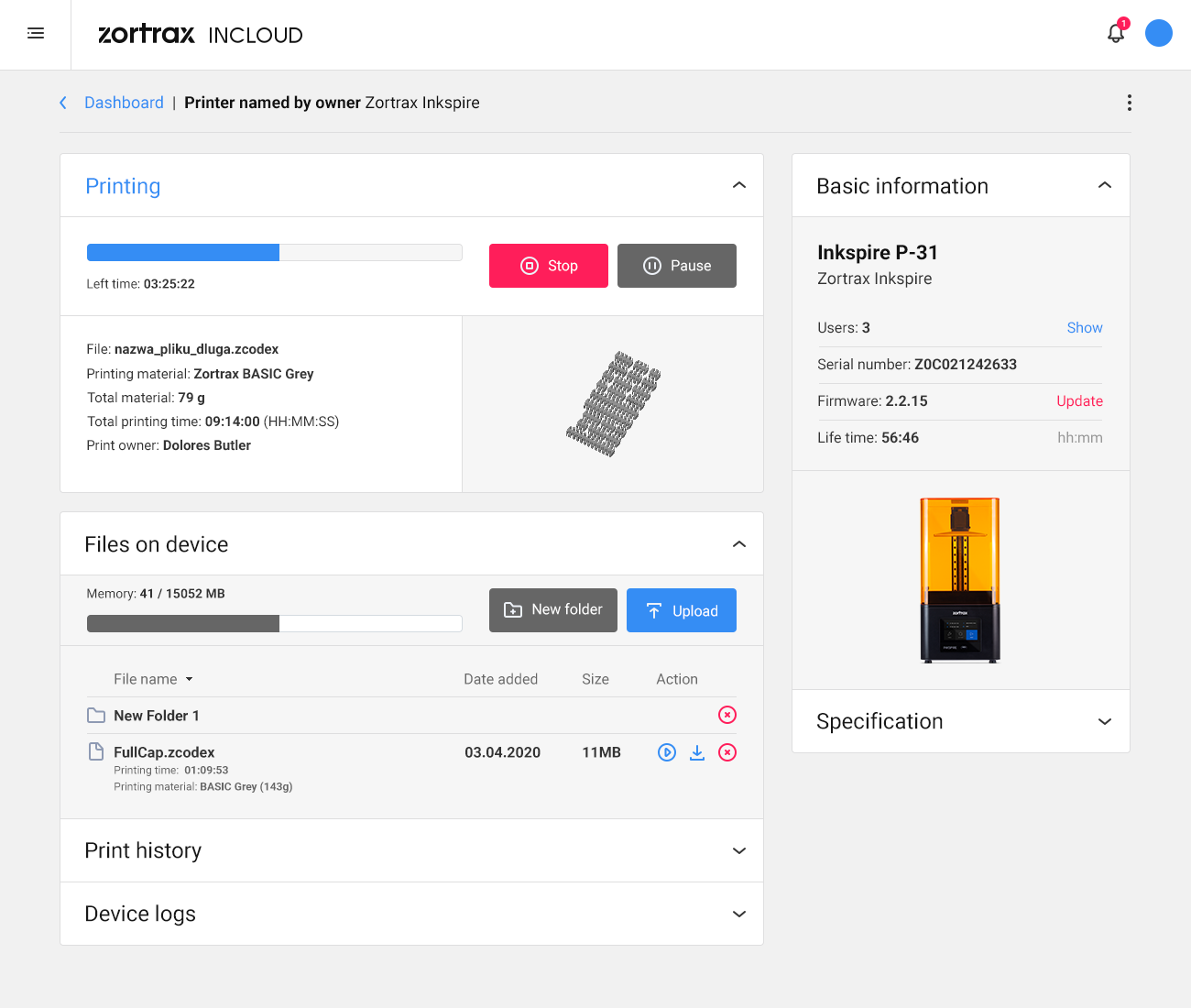A screenshot of the Zortrax Cloud interface, specifically for the Zortrax Inc. Spire 3D printer, displaying detailed printer and file information on a light gray background. On the left side of the dashboard, it showcases the printer named "Zortrax Inc. Spire" with a blue "Printing" status inside a box. The progress bar is approximately halfway filled, indicating ongoing printing. Below this, there's a file name, the printing material "Zortrax Basic Gray", total material usage of 79 grams, total printing time, and the print owner, Dolores Butler. The interface also includes a stop and pause button, and a left time indicator reading "03:25:22".

Beneath the printing information, another section titled "Files on Device" shows 41 out of 15,052 megabytes of memory used, with options to create a new folder or upload files. It lists two file names and provides access to print history and device logs.

On the right side of the page, a segment labeled "Basic Information" features the printer identification "Inc. Spire P31" and the model name "Zortrax Inc. Spire". It lists the number of users as 3, the serial number, firmware version, and a red update indicator. The lifetime usage is shown as 5646. Below this section, there's an image resembling an ink cartridge followed by the word "Specification".